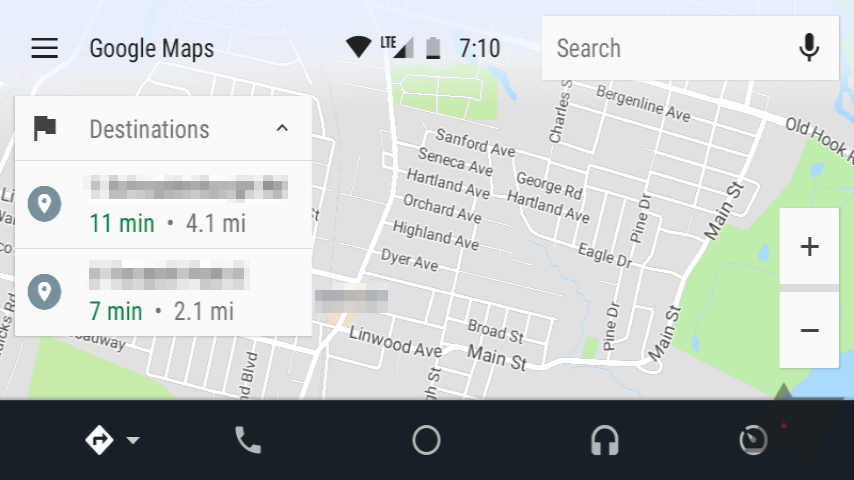The image depicts a detailed digital map interface with various elements and annotations. 

At the bottom, there is a control bar displaying icons for "Phone," "Circle," "iPhones," and a meter indicator. The top left corner features several symbols including a hyperlink icon, Google Maps, full WiFi signal, LTE connectivity, a battery icon showing "71%," and a search bar accompanied by a microphone icon. 

In the extreme left, there's a vertical rectangle marking flags and points of interest, such as destinations marked with a pin. The map details a route, indicating travel times and distances: "11 minutes, 4.1 miles" and "7 minutes, 2.1 miles." 

Several street names are visible within the map, including Sanford Avenue, Seneca Avenue, Heartland Avenue, Orchard Avenue, Highland Avenue, Dyer Avenue, Linwood Avenue, Main Street, Pine Drive, and Old Hook Bergenland Avenue. Additionally, there's a key location marked with "Charles."

Parts of the map show diverse color segments, including green areas representing grass or parks, gray areas indicative of urban or built-up regions, and a blue section in the bottom right signifying water. The streets are predominantly white, with multiple street names labeled clearly for navigation.